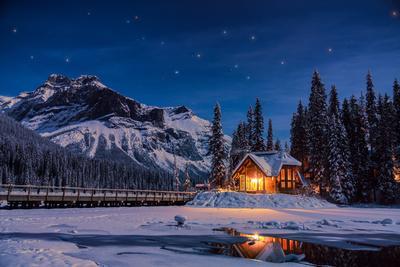This small yet intricate piece of artwork portrays a meticulously detailed nighttime winter scene that is so realistic it resembles a photograph. The sky is a deep, dark blue, speckled with twinkling stars, perfectly capturing the essence of a clear, cold night. In the distance, a large, rocky mountain, blanketed in snow, looms majestically. Beneath the mountain, on the snowy, icy ground, stands a quaint little house nestled on a slightly elevated snowy platform. Its windows emit a warm, bright orange glow, offering a stark yet comforting contrast to the chilly surroundings. Adjacent to the house runs a long railway track, suggesting a remote, serene location intertwined with the vast expanse of nature.